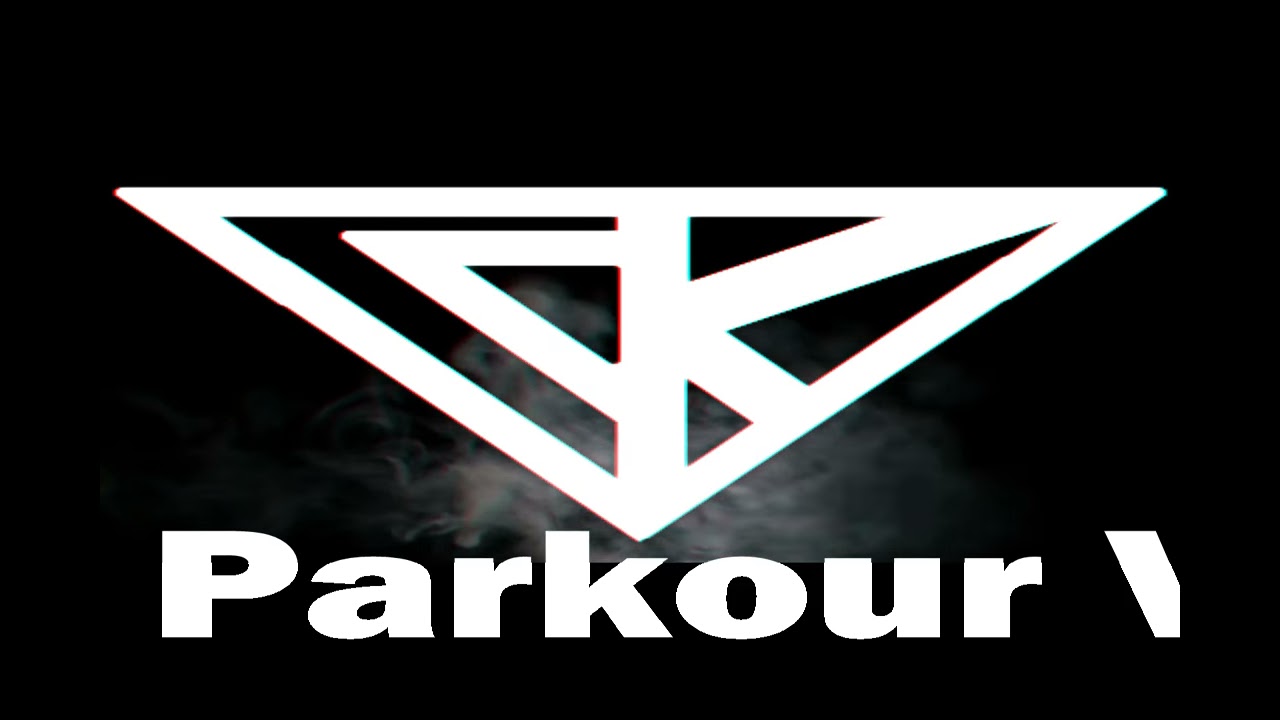In this image, the entire background is a deep black, creating a stark contrast with the central elements. Dominating the scene is a large, white triangular logo that spans nearly the entire width of the image. The logo resembles an upside-down triangle with intricate, angular designs inside it, appearing somewhat three-dimensional due to subtle red and blue outlines reminiscent of 3D effects. On the left half of the triangle, there is a design that resembles a 'C' or a left-handed triangle intersected by a bar, while the right side features a 'K' extending to the upper corner and partially down to the bottom. Behind this central logo, there is a nebulous, misty scene of smoke or clouds, adding a sense of depth and distortion to the image. Below the triangle, the text "PARKOUR" is prominently displayed in large, white block letters, with only the letter "P" capitalized. The text stretches across two-thirds of the bottom part of the image, and it appears that another word begins but is cut off by the frame, possibly starting with a "W."